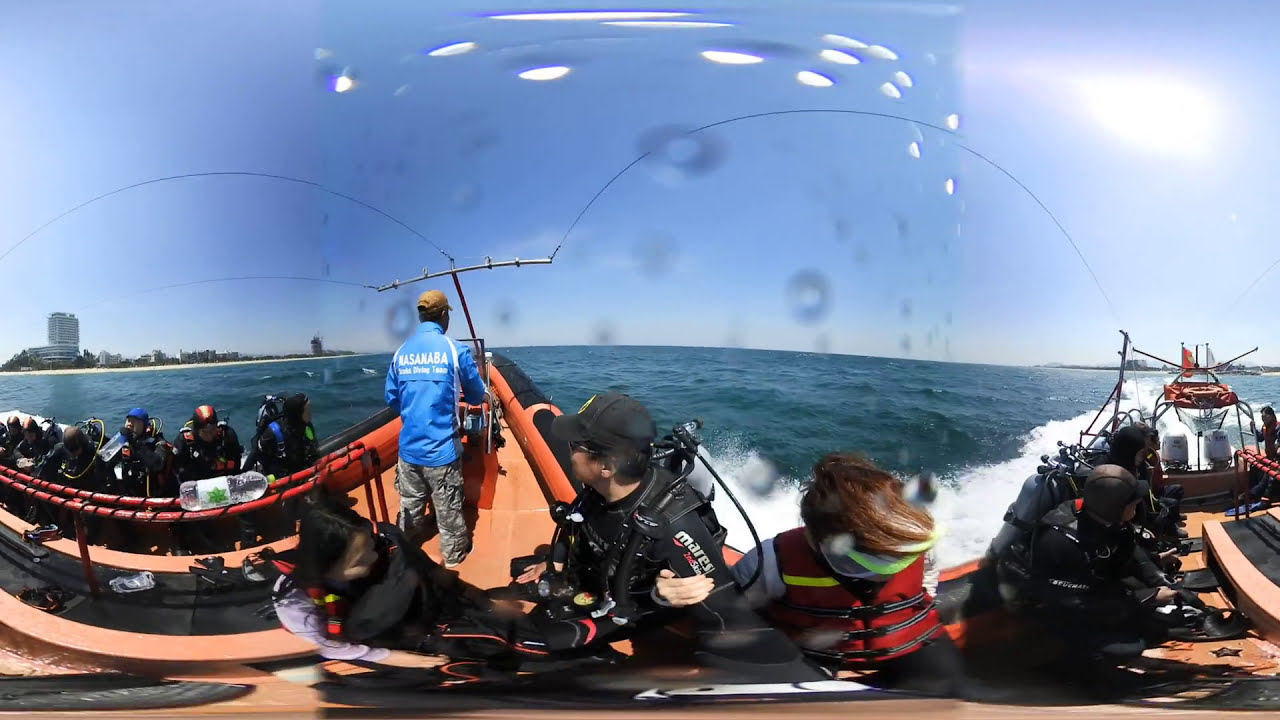The image captures a panoramic view of a boat filled with numerous people, all geared up for a scuba diving expedition. The boat's deck is vibrant orange, matched by a black railing cushioned with orange padding. Centrally positioned, though towards the left due to the panoramic perspective, a man stands behind a driver's console fixed on an orange pedestal adorned with multiple silver knobs. He is clad in grey camouflage cargo pants, a long-sleeve blue jacket featuring white text and stripes, and a tan baseball cap. Surrounding him, passengers are either seated or standing on the orange deck, each equipped with scuba diving gear, life vests in red or black, and various underwater breathing apparatus including tanks and regulators. The backdrop showcases a dazzling blue sky with the sun in the upper right corner, casting reflections on the beautiful blue water that the boat is navigating through. To the left of the image, a tall apartment building stands along the shore, framed by trees and sand. The boat appears to be trailing another vessel, indicated by the wake ahead of them. An antenna juts out from the boat’s pointed bow, further emphasizing its readiness for the aquatic adventure. The image’s 360-degree capture adds a unique curvature to the scenery, intensifying the immersive experience.